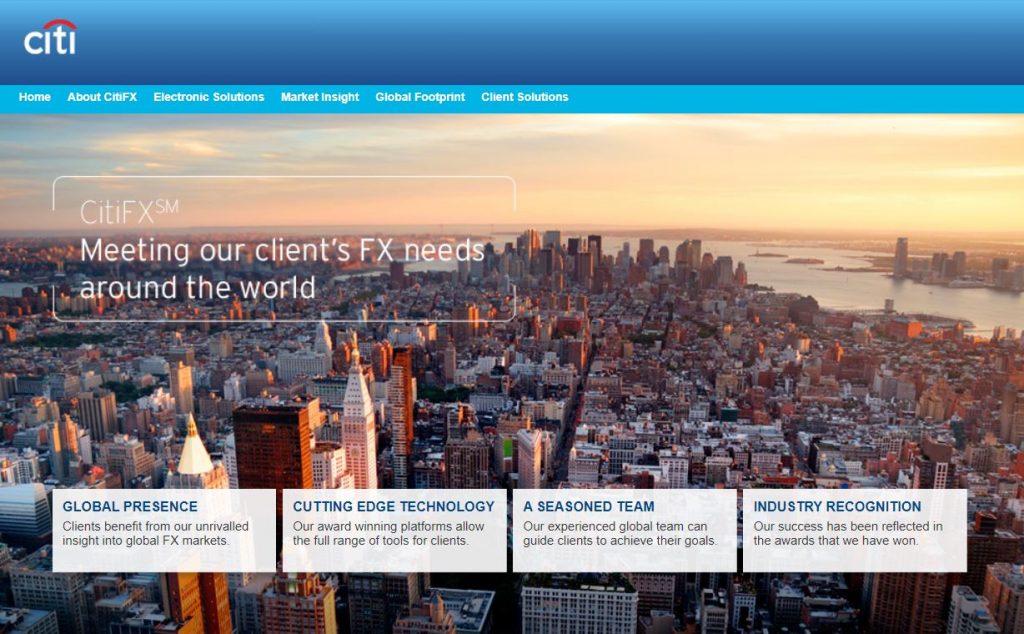A detailed screenshot of the Citi website is showcased. On the left side, the distinctive Citi logo is prominently displayed, featuring "Citi" in a white font with a red arc connecting the two 'i's. The banner across the top of the page has a gradient that transitions from medium blue to a lighter shade toward the top. Below the banner, a thin, elongated rectangular menu bar in teal blue with white font presents clickable options including: Home, About Citi, FX, Electronic Solutions, Market Insight, Global Footprint, and Client Solutions.

The central area of the screenshot is dominated by an impressive aerial view of a cityscape, likely New York, characterized by densely packed high-rise buildings, numerous roads, and water bodies surrounding the urban core with additional land extending beyond the water. Overlaying this striking image is the text "Citi FX SM Meeting Our Clients' FX Needs Around the World" in a white font, enclosed within a semi-transparent rectangular shape with rounded edges. The design and layout effectively blend visual appeal with navigational functionality, reflecting Citi's commitment to global financial solutions.